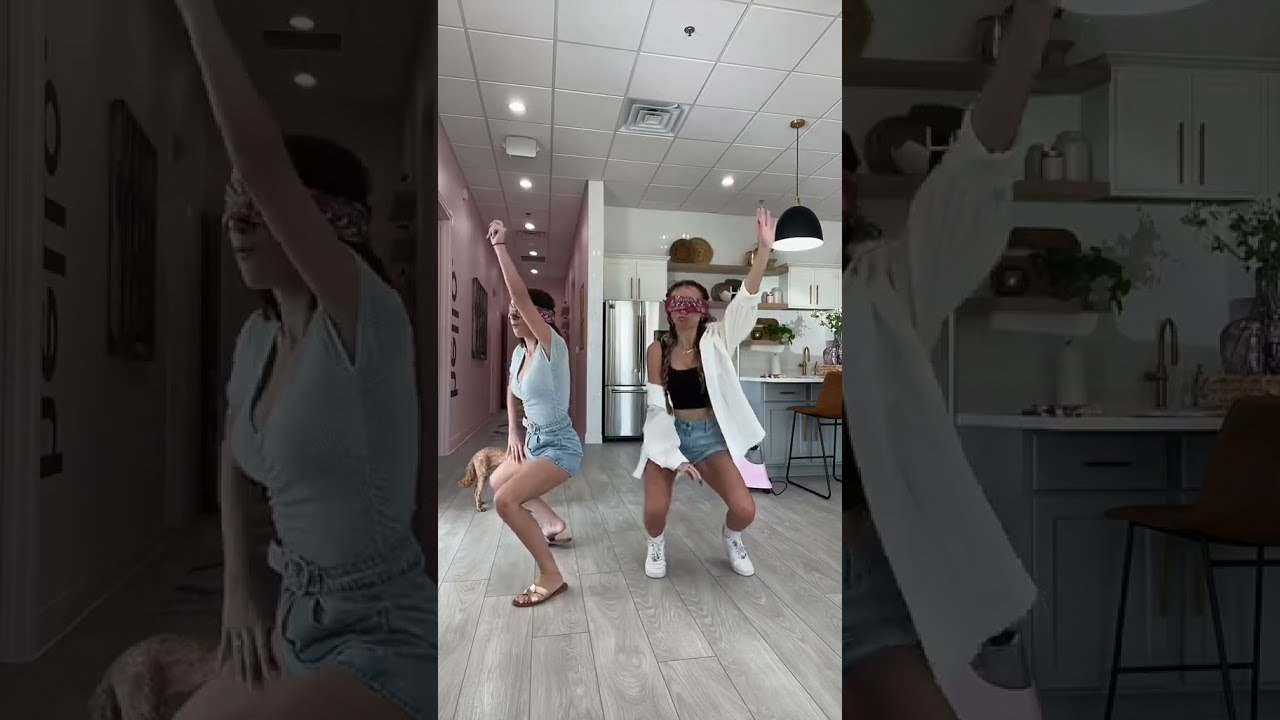In this image, two young women, seemingly in their late teens or early twenties, are captured mid-dance in what appears to be a kitchen area. The girl on the left is wearing a short gray shirt, denim shorts, and flip-flops, and she is squatting with her left arm raised. Her hand is open. The girl on the right, donning a white jacket over a black tank top and sneakers, is also squatting with one arm raised, her hand closed. Both have bandanas blindfolding their eyes, adding an element of playful mystery. The kitchen backdrop includes a table with chairs, a refrigerator, and shelves or cabinets. A pink hallway behind them leads to another part of the house, lit from above, with a decoration reading "hello" vertically on the wall. A small dog is partially visible, peeking out near the left girl's feet. The central image is flanked on either side by enlarged, darkened versions of the same scene, adding a dramatic border to the composition.